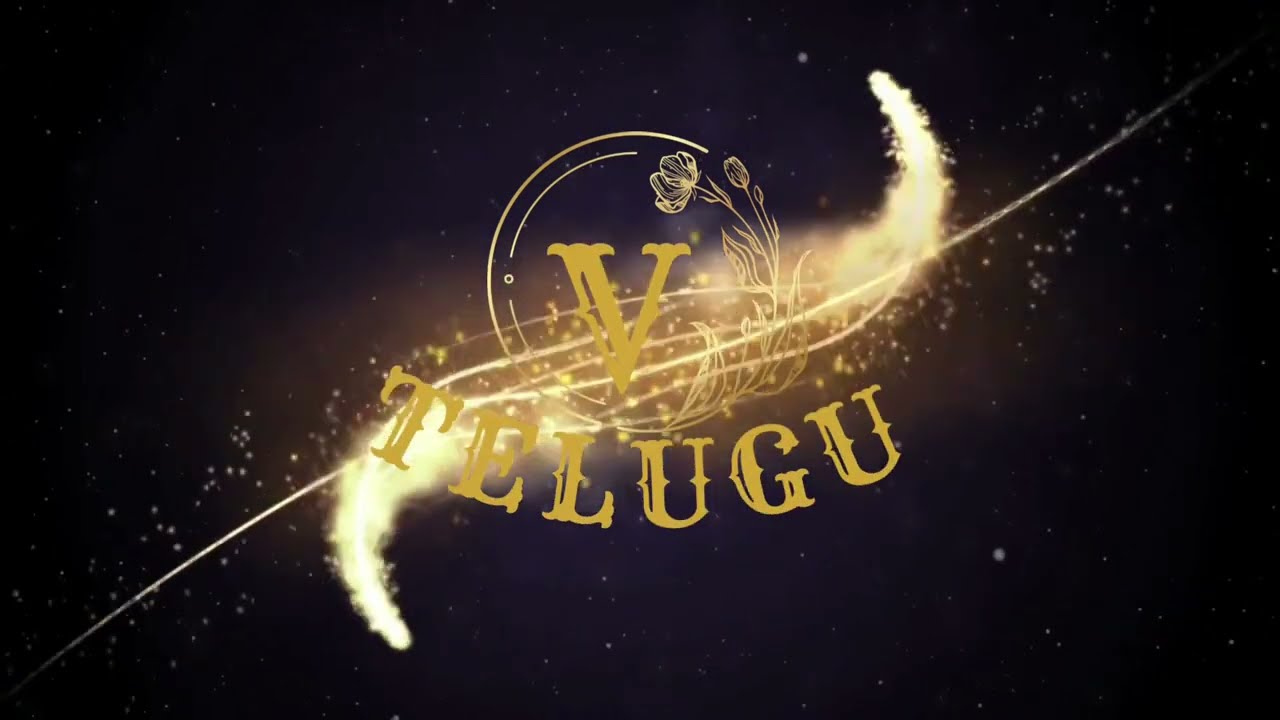This image features a rectangular, landscape-oriented design with a predominantly black background, accented by white specks representing stars, reminiscent of a starry night sky. The central logo stands out against a dark backdrop, slightly illuminated by a subtle bluish tint in the middle. A thin, bright line stretches diagonally from the bottom left to the top right, resembling a shooting star or a firework streak, which intersects the logo at its center.

At the heart of the image is a circular emblem. The right half of the circle is intricately formed by a stylized vine, complete with a tall flower, its stem, and detailed leaves extending inwards towards the circle's core. Sparks and bright yellowish trails evoke a firework effect, flaring out from the top right and top left edges of the circle, creating dynamic movement around the logo.

Prominently displayed in the center of the circle is a bold, yellow "V," designed with squared-off, blocky edges. Directly below the "V" are the capital letters "T E L U G U," also in yellow, maintaining a similar blocky, geometric style. The entire composition combines natural and celestial elements to create a striking, vibrant visual centered on the "V" and its surrounding floral and stellar motifs.